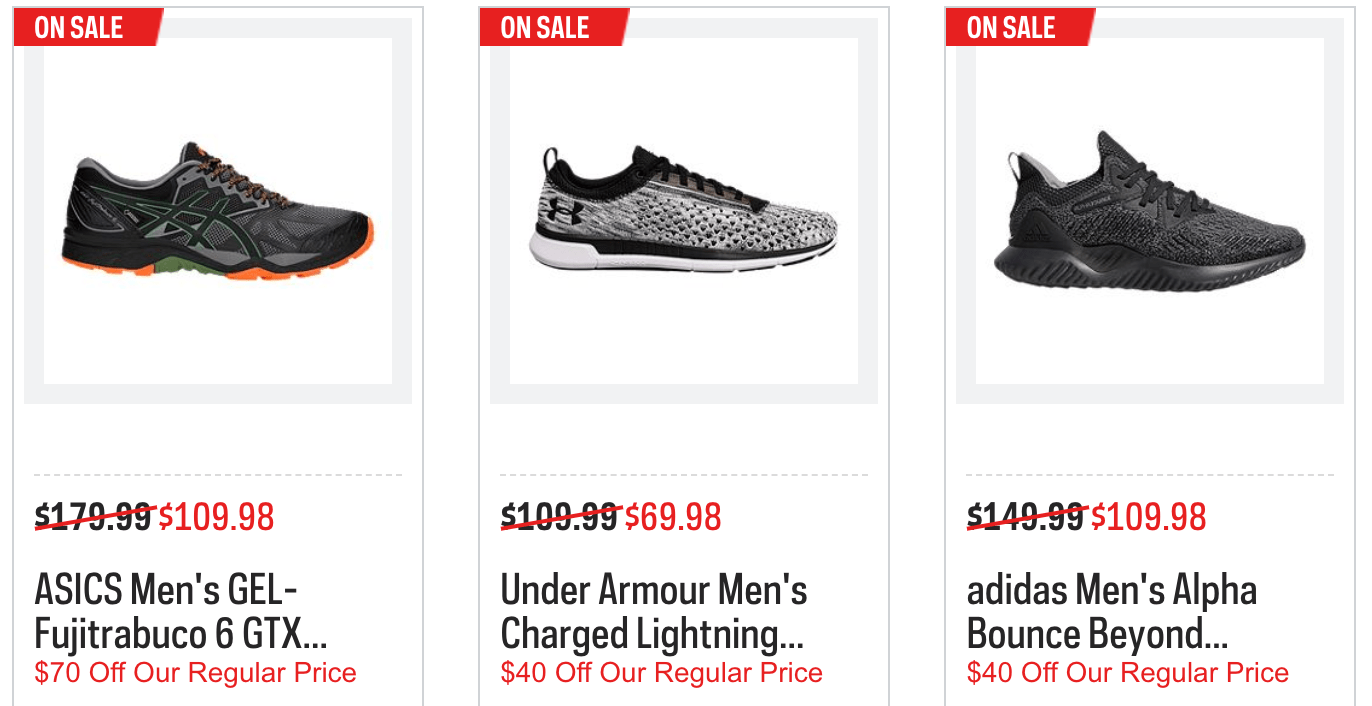Here's a detailed and cleaned-up caption for the image:

---

**Page Description: Athletic Shoes Sale**

**Left Column:**
- Against a bold red background, the words "OUR SALE" are prominently displayed in striking white text.
- Featured is a sleek black athletic shoe shown in a side profile.
- Below the image, the original price of $179.99 is crossed out in red.
- The discounted price of $109.98 is highlighted next to it in red.
- Detailed Information: "Asics Men's Gel-Fuji Trabuco 6 GTX" offering a substantial discount of $70 off the regular price.

**Center Column:**
- Titled with "ON SALE" at the top.
- Showcases another athletic shoe aimed at active individuals.
- The previous price of $109.99 is visibly crossed out in red.
- The new tempting price of $69.98 is marked in red beside it.
- Detailed Information: "Under Armour Men's Charge Lightning" available at a $40 discount from the regular price.

**Right Column:**
- Aligning with the theme of sales, "ON SALE" is written at the upper section against a red background.
- Pictured is a dark-colored athletic shoe from a side angle.
- The old price of $149.99 is struck through with a bold red line.
- The new, reduced price of $109.98 stands out in red next to it.
- Detailed Information: "Adidas Men's AlphaBounce Beyond" now at a $40 reduction from the regular price.

---

This caption provides a clear, detailed, and structured overview of the items and their prices, making it easier for the reader to understand the sales promotion.